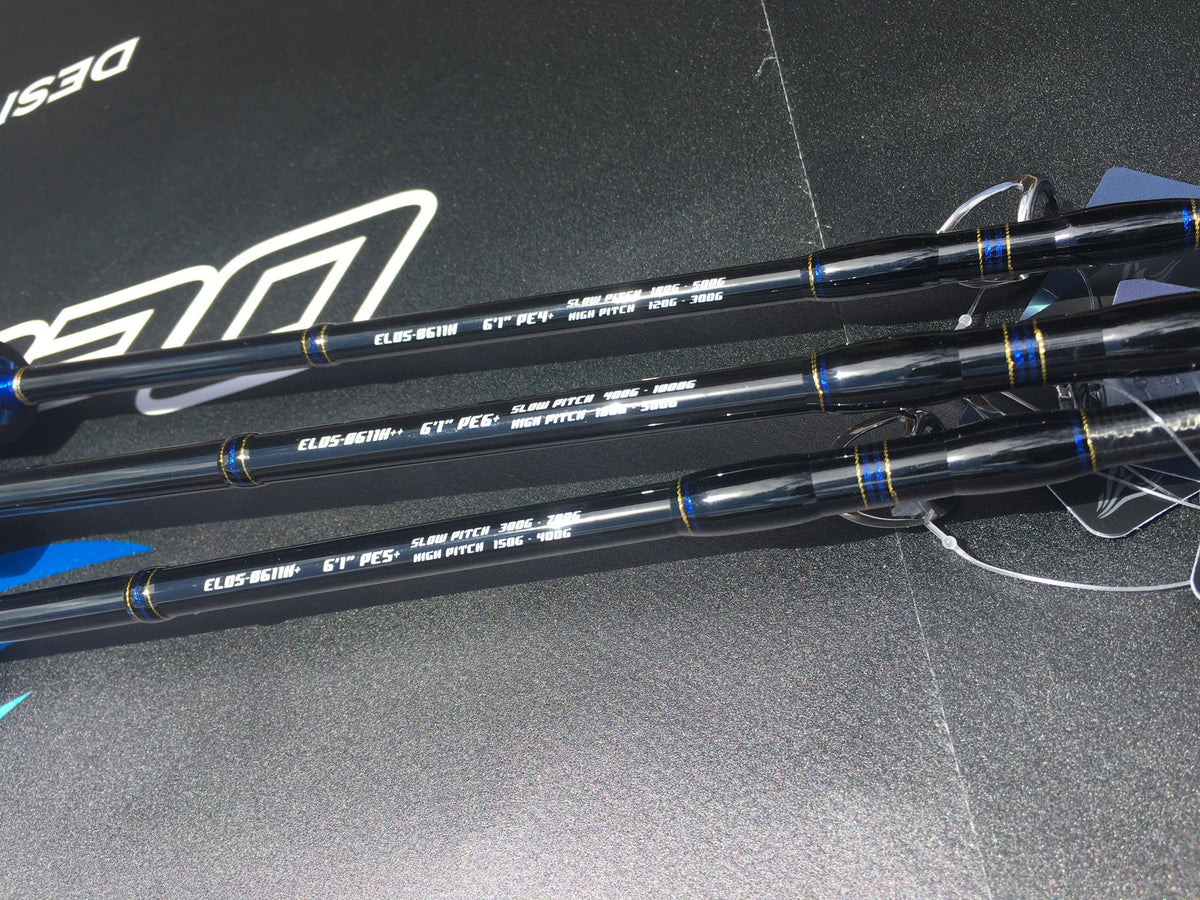This image features a trio of sleek black objects laid out parallel to each other on a background that matches their matte, black finish. These backgrounds appear to be either high-quality canvas, leather, or another textured material that complements the objects. Upon closer inspection, the items resemble arrows used for archery, distinguished by the small, plastic nock sections at their ends. Each arrow is detailed with a color scheme of blue, gold, and black, and adorned with various pieces of text. The inscriptions include phrases like "slow pitch," "high pitch," and measurements such as "6 feet 1 inch," and "P-E-G." These annotations hint at specific characteristics or specifications related to their use or design, possibly indicating range or type of arrow. The photograph is centered on the arrows, providing a detailed view but leaving some details to the imagination.